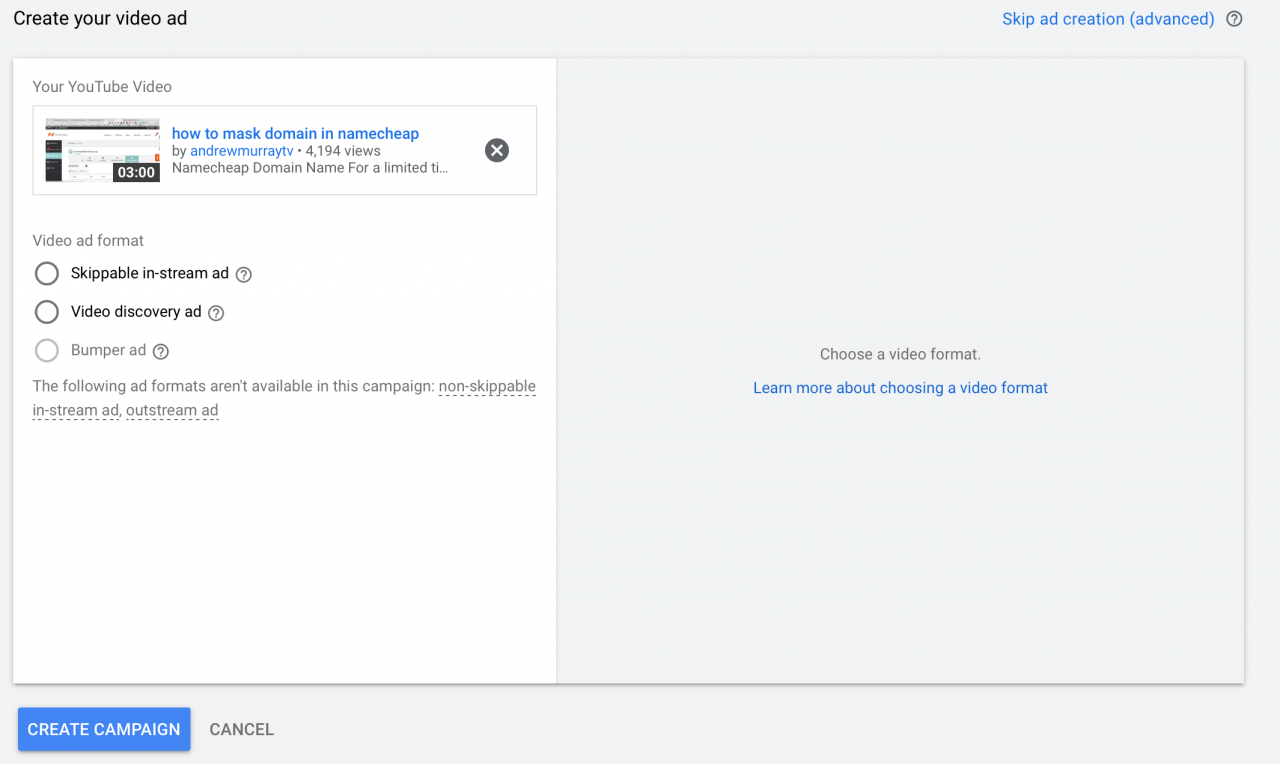The image features a user interface for creating a video ad, set against a gray background. In the upper left corner, black text reads "Create your video ad." To the right, blue text displays "Skip ad creation (Advanced)." Below this, there is a black-outlined circle containing a question mark.

Prominently in the center, a large rectangular area is divided into two sections. The left section is slightly smaller and displays a YouTube video thumbnail. The thumbnail shows a paused YouTube video with a timestamp of "03:00" in a black box at the bottom. To the right of this thumbnail, the title and details of the video are visible: "How to Mask Domain in Namecheap" by AndrewMurrayTV, with 4,194 views. The description is partially visible: "Namecheap domain name for a limited TI..."

Adjacent to the video thumbnail, a black circle with a white "X" indicates a close button for an element. Below this section, the text "Video ad format" is displayed prominently. There are three options listed:

1. An open circle labeled "Skippable in-stream ad" with an adjacent circle containing a question mark.
2. Another open circle labeled "Video discovery ad" with a corresponding question mark circle.
3. A grayed-out circle labeled "Bumper ad" with a nearby question mark circle.

The design is intended to guide the user through the process of creating or selecting a type of video ad for YouTube.